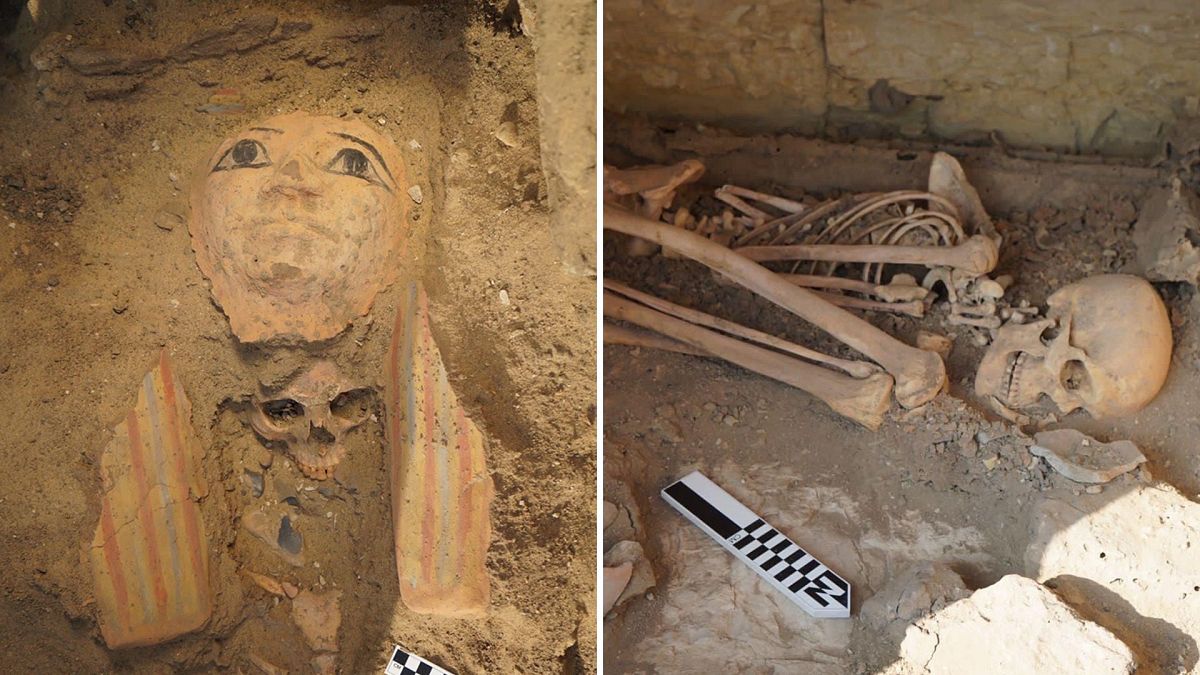The image consists of two photographs taken at an archaeological excavation site. On the left side, the photo captures part of a mummy's tomb excavation, revealing a sarcophagus mostly covered in sand. Visible details include the head and portions of the headdress of the sarcophagus. Underneath the chin of the sarcophagus head lies a human skull. The right side photo is set within a similar catacomb or tomb environment and features a jumbled human skeleton piled together. Both photos are equal in size and depict the careful excavation of these ancient human remains, surrounded by sandy dirt. A checkered marker, often used in archaeological digs, can also be seen next to the skeletons, aiding in the documentation and analysis of the site.